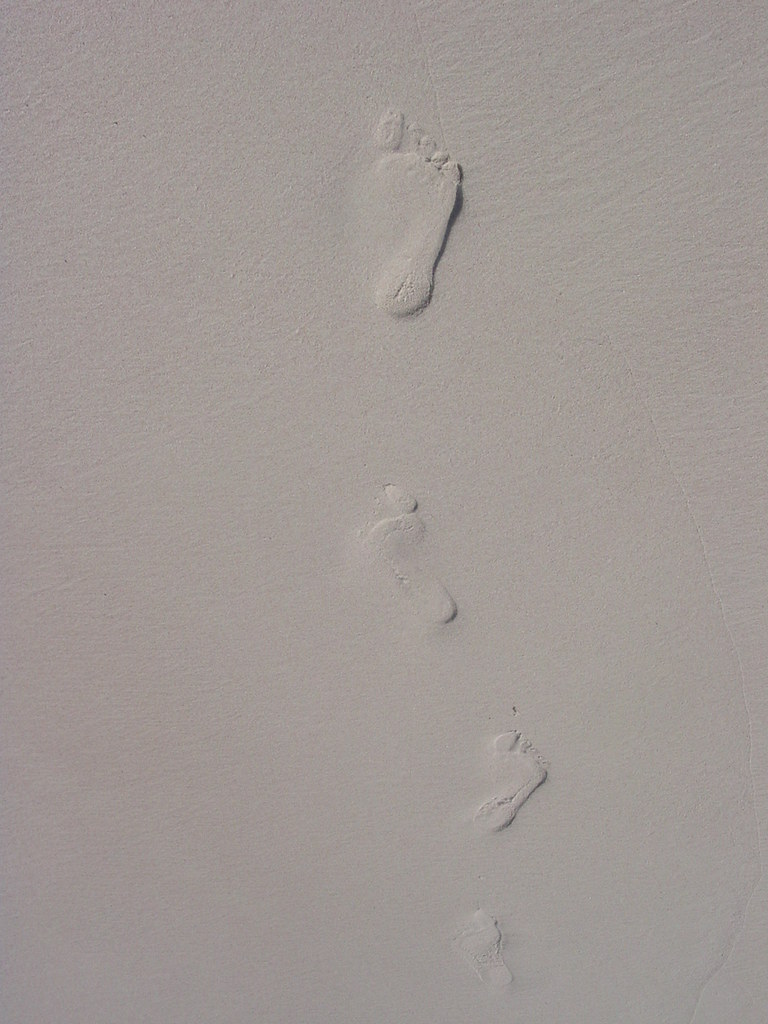This close-up image depicts a textured gray surface that resembles either fine beach sand or cement, likely more like cement, based on its grayish silver color. The surface is smooth without any impurities like rocks or foreign objects. The most striking elements are the series of four footprints progressing from the bottom to the top of the image. 

Beginning at the bottom, there is a tiny footprint, followed by progressively larger ones as you move upwards. Positionally, they alternate feet: a left footprint at the bottom, followed by a right, then a left again, and finally, a large right footprint at the top center. Each footprint shows clear details of the foot, heel, and toes, and the indentations create distinct shadows. The footprints don't lie flat but appear slightly raised from the sandy or cemented ground, adding depth to the otherwise plain background. Despite an outdoor setting that could be a beach or a driveway, there's no additional context provided in the image.